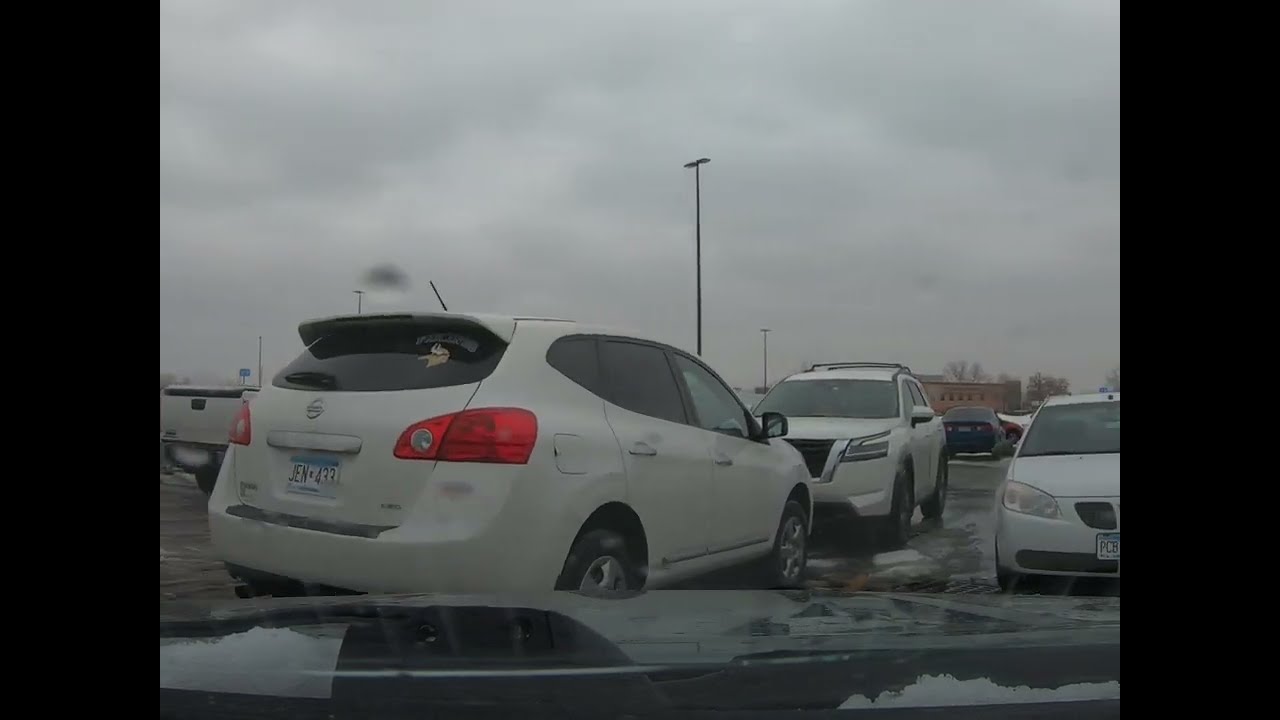In this detailed photograph, a gray, cloudy sky looms over a snow-covered, wet parking lot viewed from the driver's side of a car, looking out through the windshield. The scene features several parked vehicles, primarily SUVs, including two white SUVs, a white truck, a distinct white car, and a distant blue car. The dirty snow covers the black asphalt, intermittently clean and sullied by vehicle traffic. A Minnesota Vikings decal on one SUV hints at the location being Minnesota. In the background, a brick building peeks through a cluster of trees. The parking lot is also punctuated by poles with lights, reinforcing the overcast, wintry atmosphere.